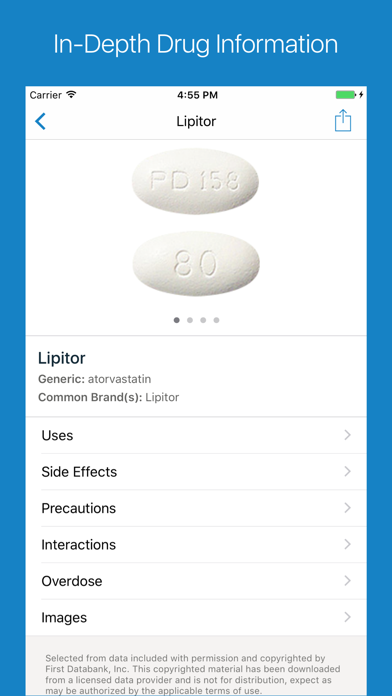The image depicts a smartphone screen displaying detailed drug information. The outermost border of the screen is a royal blue rectangle. Moving inward, there is a central white rectangle. At the top of the blue border, "In-depth drug information" is written in white text. Within the white rectangle, the screen status bar shows the word "carrier" at the top left, the time "4:55 p.m." in the center, and a fully charged battery icon with a green indicator on the right. 

Beneath this status bar, a blue left-pointing arrow is positioned on the left, "Lipitor" is prominently displayed in the center, and an upload button appears on the far right. As you scroll down, a high-resolution photograph of a pill is visible. One side of the pill is marked with "PD 156," and the other side shows "80." There are four navigation dots below the pill image, suggesting more pictures are available to view.

Further down, the text "Lipitor" appears as a header, followed by "generic" and common brands including "Lipitor" itself. Finally, the bottom section includes labelled tabs for additional details: uses, side effects, precautions, interactions, overdose, and images.